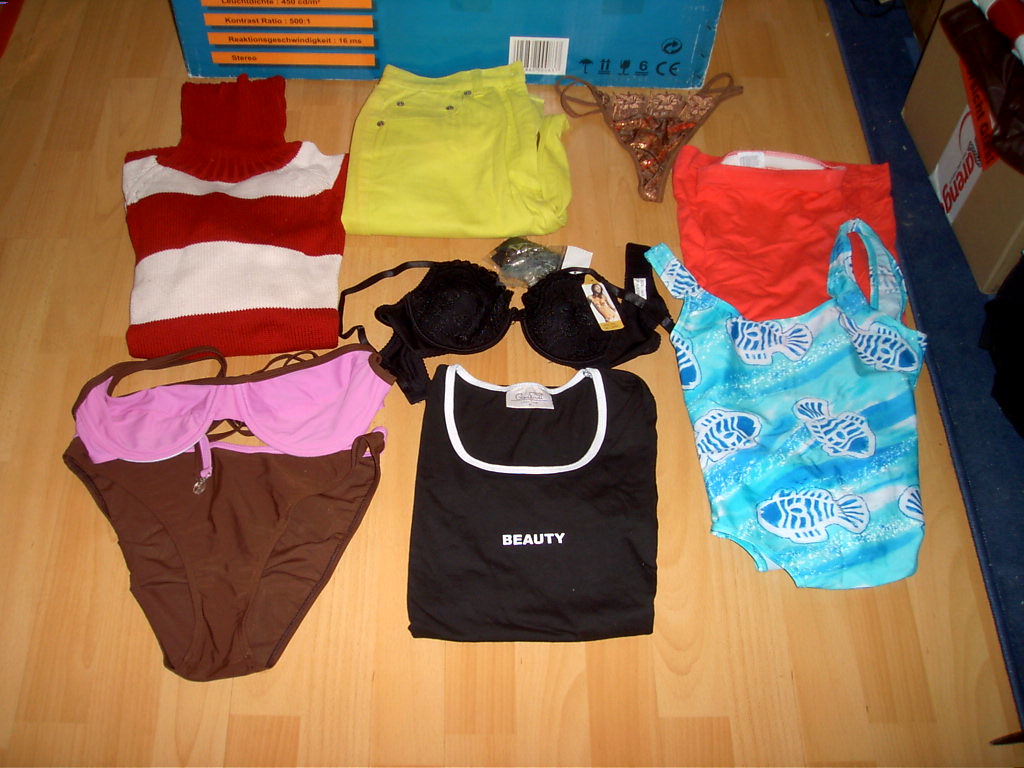This photograph captures a neat arrangement of various clothing items spread across a light brown wooden table. In the top left corner, there is a striking red and white striped turtleneck sweater. Moving right, you find a pair of neatly folded yellow shorts. Next, a dazzling pair of gold sequined bikini-style underwear catches the eye. 

On the bottom row, starting from the left, we see a stylish pink bikini top with brown straps, paired with brown bikini bottoms. Adjacent to it is a black bra, still with its white and gold tag attached. Just below the bra lies a black t-shirt with a white scoop neckline and the word "BEAUTY" emblazoned in bold white capital letters. To the far right, a colorful and playful ensemble features a red swimsuit bottom coupled with a blue top adorned with fish images.

Additional elements to note include a white and red-labeled box and a black bag resting on the right-hand side of the table, along with a blue-colored rug peeking from the same side, enhancing the overall composition of the scene.